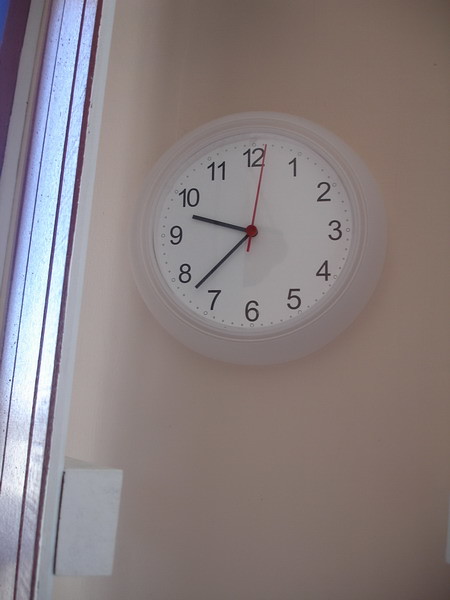This image showcases a white circular wall clock mounted on a white wall. The clock displays standard numerical digits from 1 to 12, with black hour and minute hands, and a red second hand. The time on the clock reads 9:38, almost 9:39. Adjacent to the clock, on the left-hand side of the frame, is a partially visible wooden panel door, characterized by a natural wood stain on the front and a white backing strip. The image also includes a small, indistinct reflection on the clock, and no other visible text.